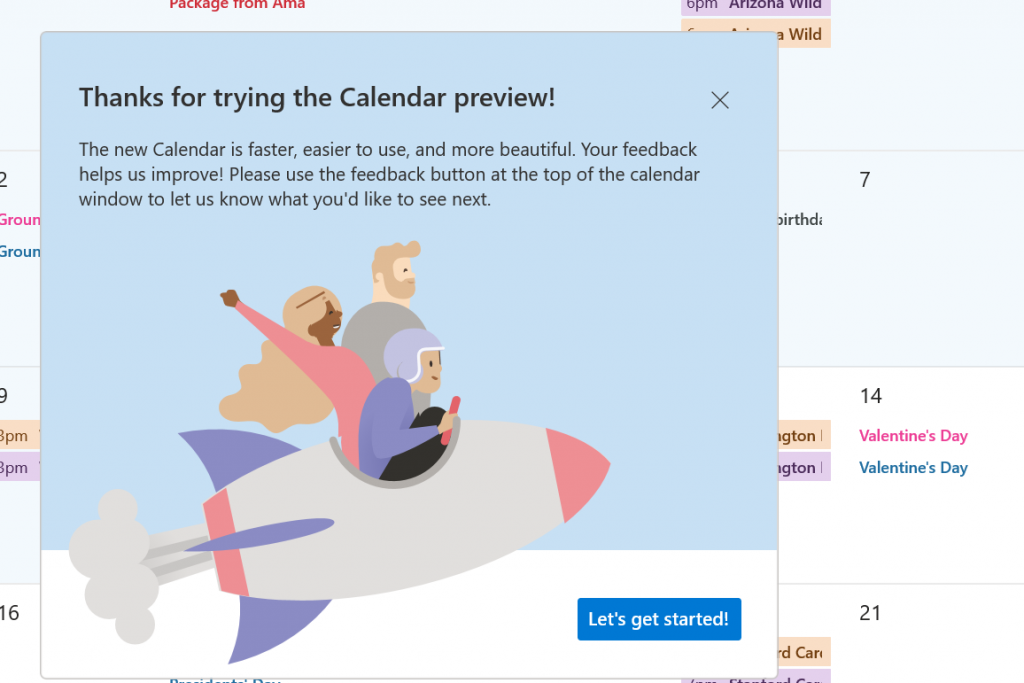This image features a vibrant and dynamic preview screen from an application, presented in a colorful and engaging layout. The screen is set in a landscape orientation with a distinct pop-up window in the foreground. This square-shaped pop-up has a light blue background occupying the top 80% and a white background at the bottom. 

At the top of the pop-up, in bold black font, a message reads, "Thank you for trying the calendar preview!" followed by an exclamation point. Below this, a subheading explains, "The new calendar is faster, easier to use, and more beautiful. Your feedback helps us improve. Please use the feedback button at the top of the calendar window to let us know what you'd like to see next."

Central to the pop-up’s imagery is a whimsical illustration of three individuals inside a rocket ship. The rocket, gray with a red tip and tail, ejects a cloud of smoke and features purple fins. The three passengers include a blonde-bearded man in a gray shirt, a blonde-haired woman in a pink dress, and another woman wearing a purple helmet and shirt with black pants, steering the ship with a red wheel.

Beneath this illustration, a long rectangular blue button bearing the text "Let's get started" in white invites users to proceed. In the background of the image, a calendar is partially visible. While the details are somewhat blurred, "Valentine's Day" is clearly marked on the 14th.